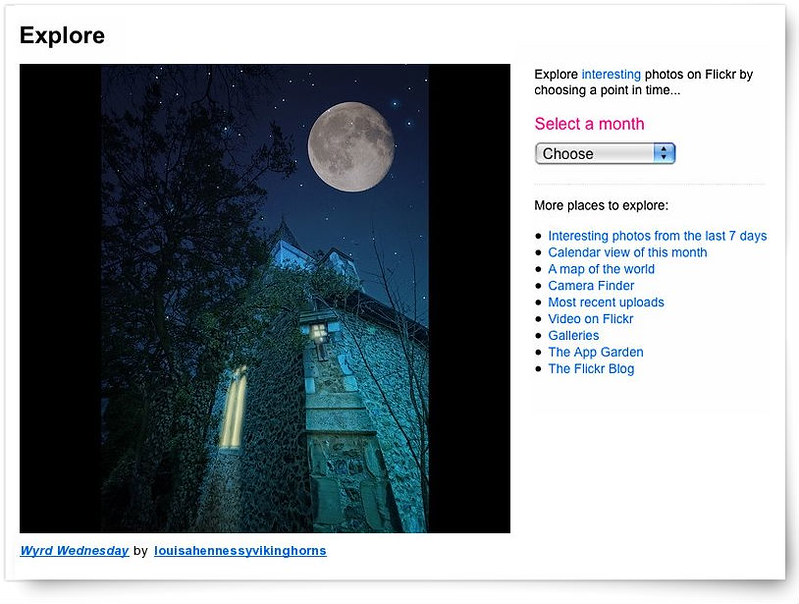The image appears to be a screenshot of a webpage, likely from Flickr, with a focus on exploring photos. Dominating the scene is a nighttime photograph of an old cathedral house, partially covered in ivy, set against a dark, starry sky with a large, full moon positioned in the upper right corner. A large tree can be seen beside the house, with one of its windows emitting a faint yellow glow, contributing to a somewhat eerie, haunted house atmosphere. The image is placed slightly to the left of the composition. 

At the top left of the screen, the word "Explore" is prominently displayed in black text. Below it, the text "Weird Wednesday by Louisa Hempsey-Vikinghortz" is written, possibly identifying the photograph or theme. On the right side of the image, there's a column of clickable blue text, offering various options for exploration: "Choose a point in time" with a drop-down menu for selecting a month, "More places to explore," "Interesting photos from the last seven days," "Calendar view of this month," "A map of the world," "Camera finder," "Recent uploads," "Video on Flickr," "Galleries," "The App Garden," and "The Flickr Blog." The background of the webpage is primarily white, with additional colors including black, dark blue, gray, light blue, and pink. 

Overall, the page appears to be a well-organized and interactive interface designed to encourage users to explore a wide array of photographs and media.